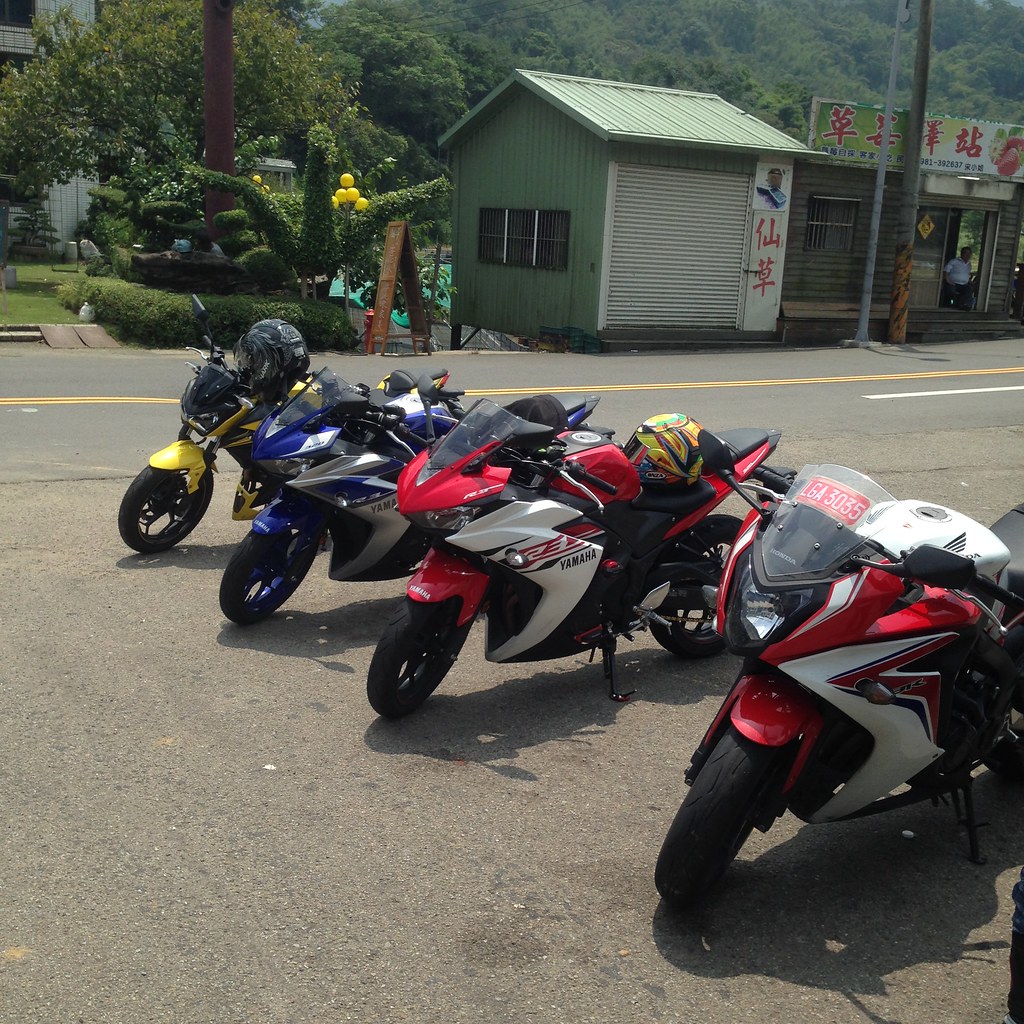This outdoor, daytime photo captures four vibrant sports motorcycles parked in a row on a paved surface, bordered by a road with a yellow stripe. The motorcycles, aligned in a diagonal line from the lower right corner to the left background, include two red motorcycles with white stripes, one blue with silver stripes, and one completely yellow motorcycle. All appear to be brand new Yamaha models. Notably, the first red motorcycle displays a helmet on its handlebars, and another yellow-tinged helmet rests on the backseat of the third bike. The first bike's license plate shows the number 3035.

The background reveals an Asian, possibly Japanese, residential area with notable features such as a storefront adorned with what could be Mandarin characters, neatly trimmed green hedges shaped into various forms including a crane, and yellow round light bulbs on poles. These elements frame the scene, adding depth with multiple small structures, such as huts and shacks, a green garden, and a distant forest nestled alongside a mountainous backdrop. Sunlight from the left side casts soft shadows on the ground, enhancing the detailed, dynamic composition of the photograph.